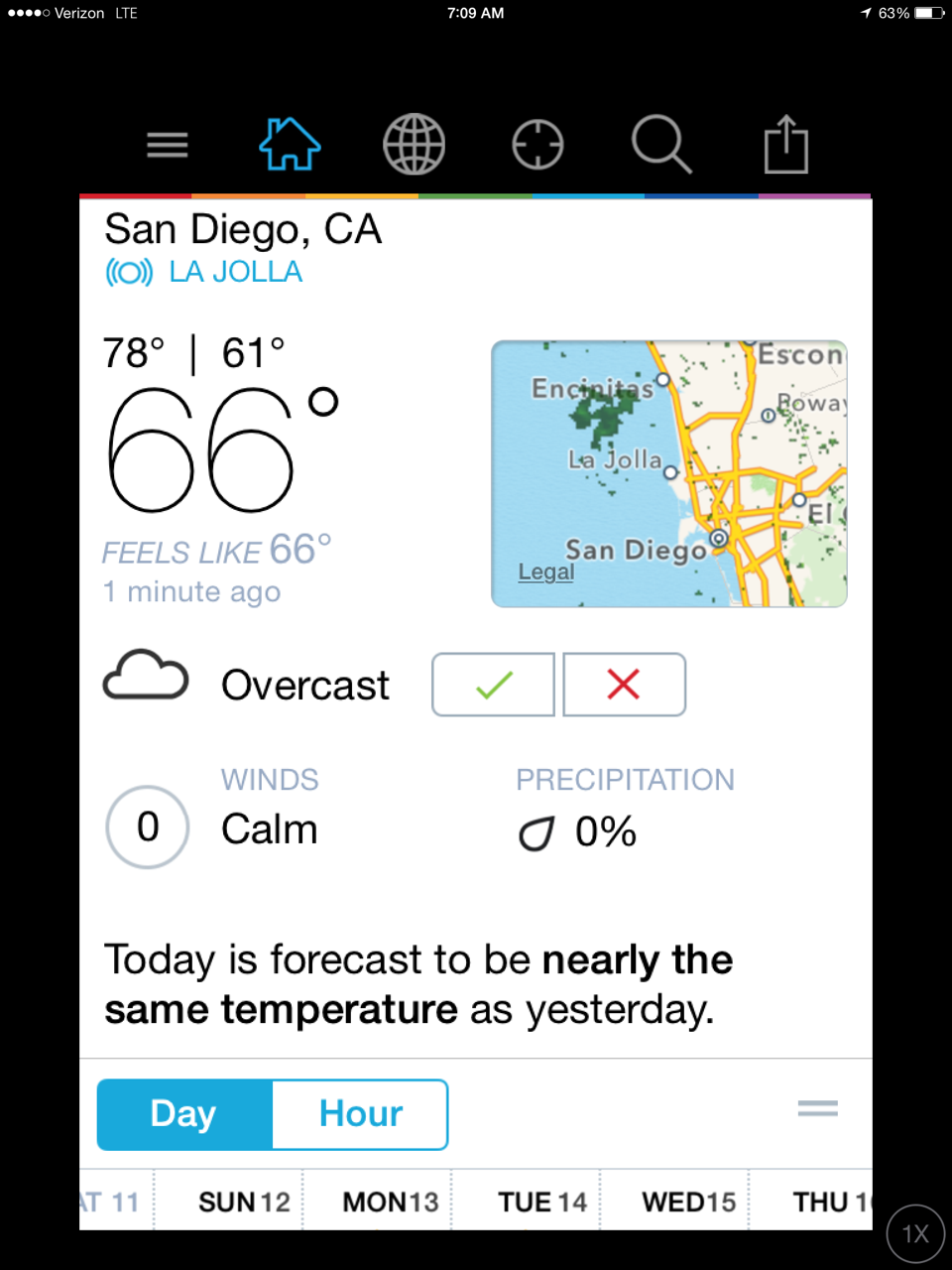San Diego Weather Forecast for La Jolla County:

- **Current Temperature:** 66°F (Feels like 66°F)
- **High:** 78°F
- **Low:** 61°F
- **Conditions:** Overcast
- **Wind:** Calm
- **Precipitation:** 0%
- **Comparison to Yesterday:** Similar temperatures expected
- **Additional Information:** An 11-day extended forecast is available.

Location Note: La Jolla is situated right along the coastline of San Diego, California.